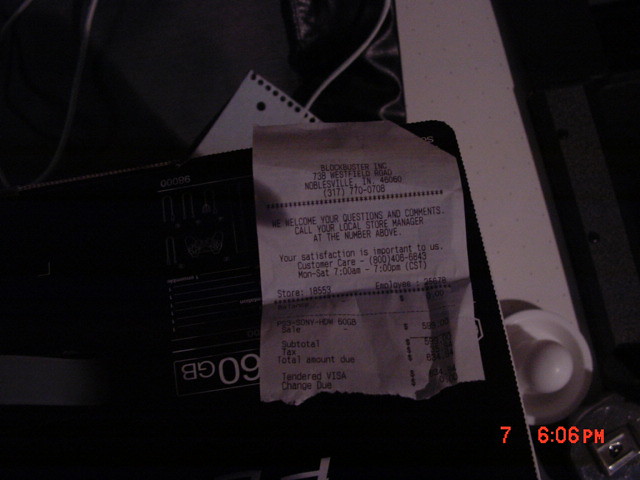In this photograph, the central focus is a prominently displayed white Blockbuster receipt printed with black font. The receipt is lying on a black folder-like object that has some white lettering on it. At the bottom of the photograph, there is a partial stamp that features the number "7" on one side and the time "6:06 p.m." 

From top to bottom, the Blockbuster receipt reveals the following details:

- The header reads "Blockbuster, Inc." 
- The address is listed as "738 Westfield Road, Noblesville, Indiana," including a zip code.
- The store's phone number is (317) 770-0708.
- The receipt indicates an invitation for questions and comments, encouraging customers to contact their local store manager at the provided phone number.
- Additionally, it lists a customer care phone number.
- Store hours are specified as Monday to Saturday from 7 a.m. to 7 p.m.
- Details of an employee number are included.
- Mention of a Sony product is present, though specific details about the item and its sale price remain partially obscured by shadows and are difficult to discern.

Overall, the image evokes nostalgia, capturing a typical transaction experience from a bygone era of video rental stores.